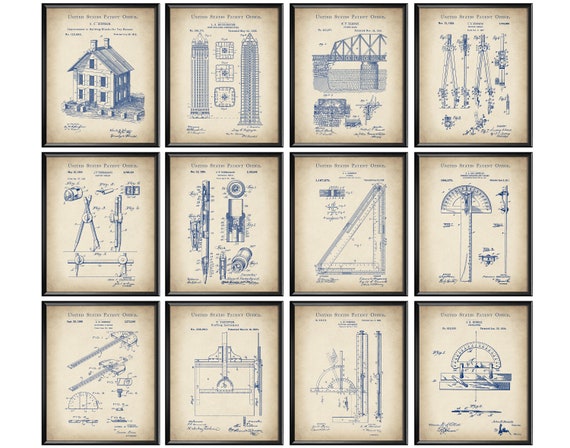The image features a tight square cluster of 12 small, extremely detailed vintage blueprints, all framed in black. These blueprints are meticulously arranged in four columns and three rows against a weathered, yellowed background, each one printed in blue ink. The top row begins with a blueprint of a house, followed by a depiction of a tall double-tower structure, and then an intricate drawing of a bridge supported by robust columns over water. The subsequent images in the first row vary in scale and detail, showing mechanical objects that are less clear.

Moving down, the second row includes diagrams of precise architectural tools: compasses, protractors, and other measuring devices used by architects. The third row continues with more detailed drawings of drafting tools, including various types of rulers and straight-edges. Each image has etched writing, enhancing their authenticity and vintage appeal. The collective arrangement of these blueprints not only highlights different architectural constructs but also the essential tools used in drafting and designing them.